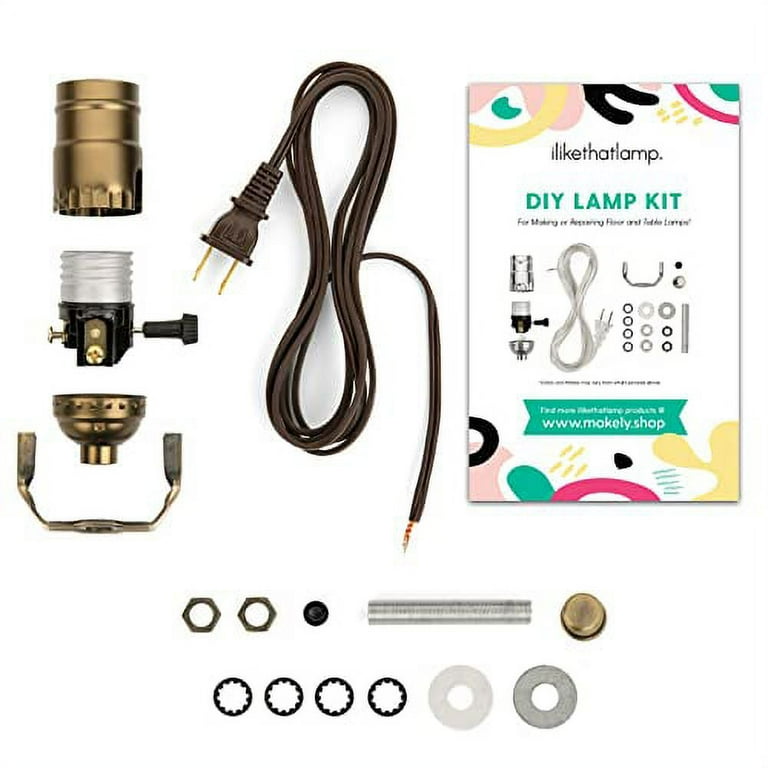This is a detailed product image showcasing the contents of an I Like That Lamp DIY Lamp Kit, neatly laid out against a simple white background. To the left, the disassembled components for the bulb fixture include a brass-colored cylinder, a white cylinder, a brass dish, a black box with a dial, and a brass Y-shaped implement. At the center lies a neatly coiled brown extension cord in a figure-8 pattern, with its copper wiring exposed and golden plugs on the left. To the right, there is a booklet with a white background, adorned with pink and yellow designs, which reads "I Like That Lamp" in black text and "DIY Lamp Kit" in blue text. Beneath this text, there is information about making the lamp and images of the kit components. At the bottom of the frame, various hardware components like bolts, screws, washers, nuts, a silver dowel, and black cogs are arranged methodically. All of these parts come together to allow you to build your own unique goldish-bronze lamp.